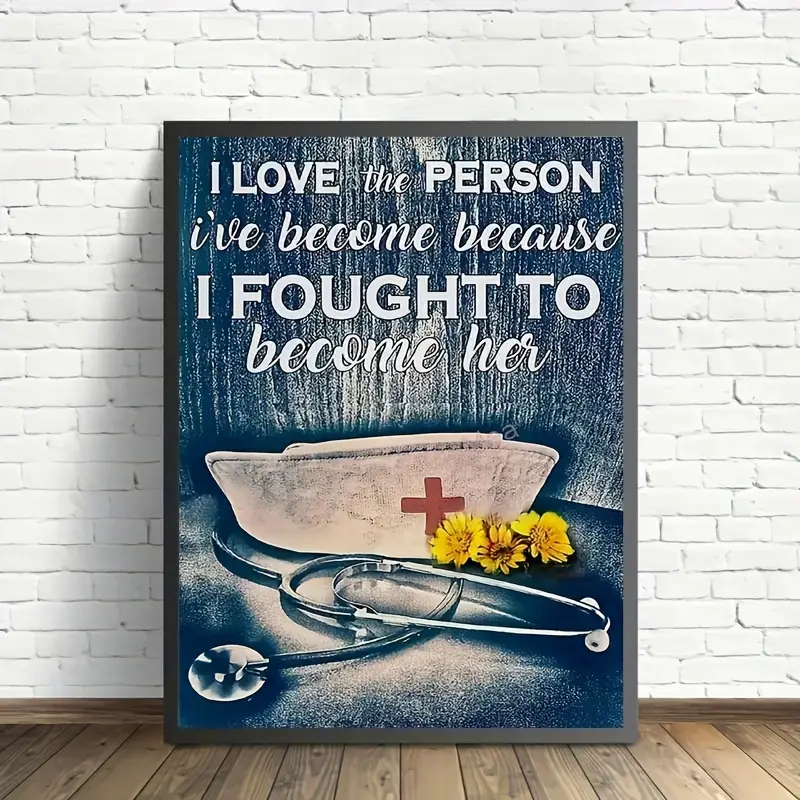The image portrays an inspirational poster with a monochromatic theme, predominantly featuring shades of black, white, and gray. Centerstage within a plain black frame, white text boldly states, "I love the person I've become because I fought to become her," mixing block letters and cursive to emphasize the message. The poster leans against a meticulously painted white brick wall, with a brown wooden floor providing a warm contrast. Placed at the bottom of the poster is an old-fashioned Red Cross nurse's hat, which stands out with its crisp white fabric and vivid red cross. Beside the hat, three yellow dandelion-like flowers and a classic black and white stethoscope add subtle touches of color and authenticity, evoking a sense of dedication and resilience. The overall aesthetic, with its muted background and vintage medical elements, exudes a timeless, heartfelt tribute to personal growth and the noble profession of nursing.